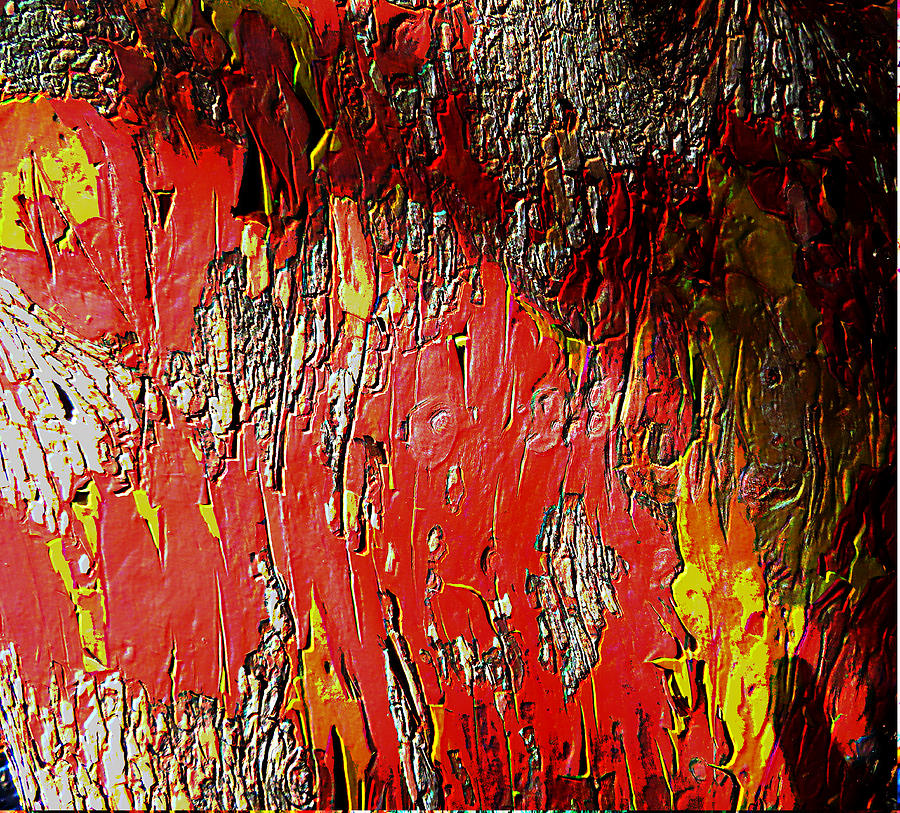The painting is an intricate abstract piece dominated by vibrant flames of light in bright reddish tones, interspersed with hints of yellow and orange. The paint is applied thickly, creating a rich texture reminiscent of weathered tree trunks with peeling bark, exposing lighter underlayers like the white spots seen throughout the artwork. The composition features heavily layered swatches of paint stretching from top to bottom, giving it a distinct textured appearance. The colors, predominantly red, darken noticeably towards the upper right corner, adding depth to the piece. This painting, a striking depiction of personal struggle, is designed to make the flames stand out, symbolizing the artist's significant journey through hardship.